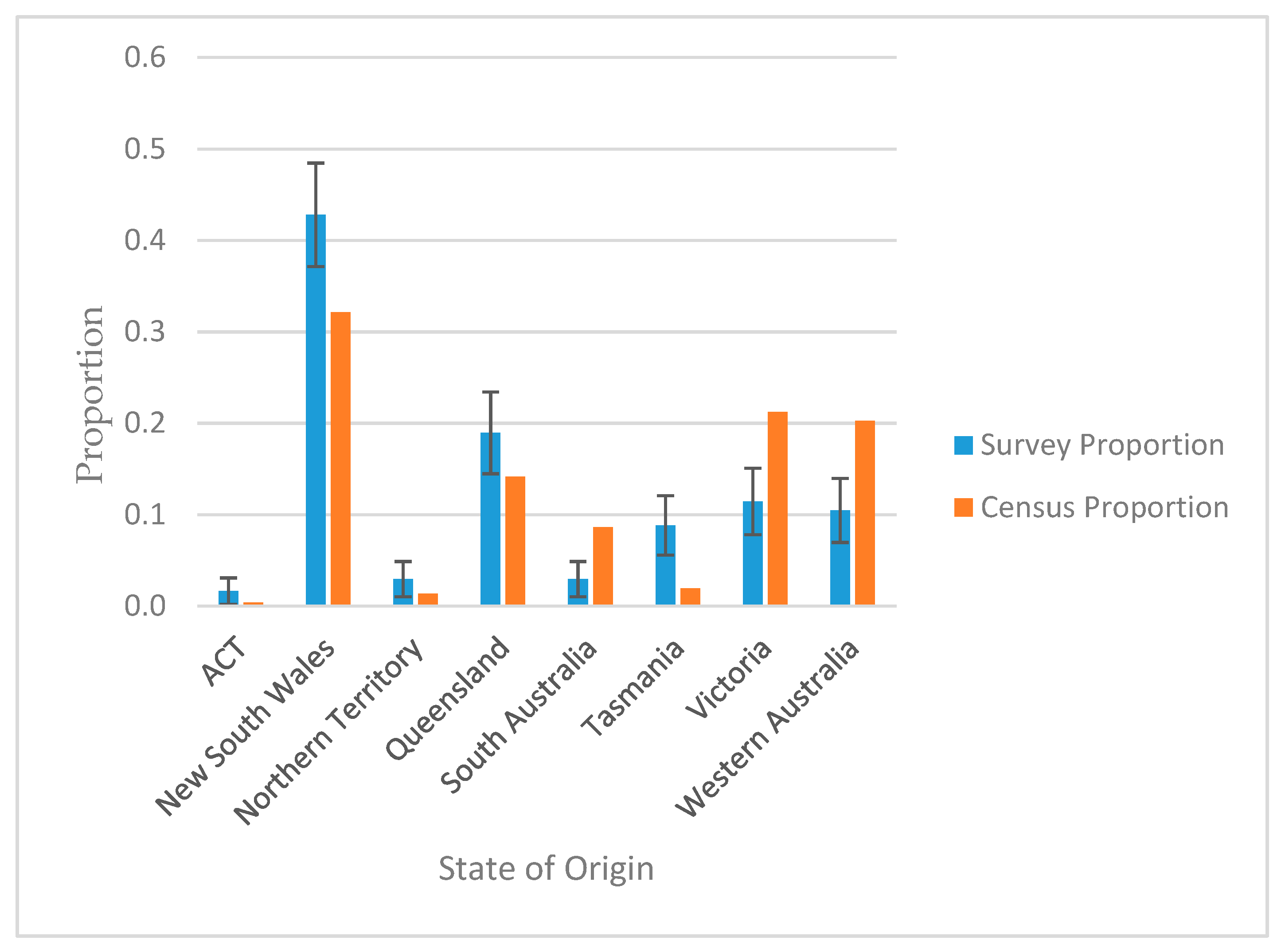This detailed bar chart compares survey and census proportions across various Australian states. The vertical axis, labeled "Proportion," ranges from 0.0 at the bottom to 0.6 at the top. The horizontal axis, titled "State of Origin," includes the states ACT, New South Wales, Northern Territory, Queensland, South Australia, Tasmania, Victoria, and Western Australia. Each state features two bars: a blue bar representing the survey proportion and an orange bar indicating the census proportion. The bars exhibit varied proportions with no apparent pattern, as some states show significantly different values between survey and census data. The chart's background is white, with black text and lighter numerical guides, and it includes horizontal grid lines for reference. There are no additional titles or explanatory text provided within the chart.